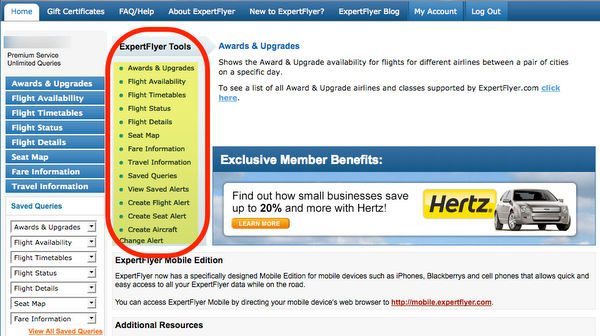Screenshot Description:

The screenshot captures a web page with a blue border extending from the left corner to the right corner, encapsulating the main navigation menu. This menu includes the items: "Home" (outlined in white), "Gift Certificates," "FAQ/Help," "About," "Expert Flyer," "New to Expert Flyer," "Expert Flyer Blog," "My Account," and "Logout."

In the left-hand column, there is a section titled "Premium Service," which boasts "Unlimited Queries." Below this title are various options listed: "Awards and Upgrades," "Flight Availability," "Flight Timetables," "Flight Status," "Flight Details," "Seat Map," "Fare Information," and "Travel Information."

Adjacent to this column, there is a section bordered in red labeled "Expert Flyer Tools." This section reiterates some previous options and adds new ones: "Awards and Upgrades," "Flight Availability," "Flight Timetables," "Flight Status," "Flight Deals," "Seat Map," "Fare Information," "Travel Information," "Saved Queries," "Create Flight Alert," "Create Seat Alert," "Create Aircraft Change Alert."

Next to the tools section, content is described under "Awards and Upgrades." It mentions the availability of awards and upgrades for flights across different airlines between specific cities on specific dates. A link is provided to see a comprehensive list of all award and upgrade airlines and classes supported by ExpertFlyer.com.

Beneath this area, there's a section labeled "Exclusive Member Benefits," highlighting potential savings of up to 20% or more for small businesses with Hertz. This section includes the Hertz logo and an image of a gray vehicle.

Further down, there is information about "ExpertFlyer Mobile Edition."

At the bottom of the page, there is another section titled "Additional Resources," which presumably offers more links and information, although specific details are not included in the given text.